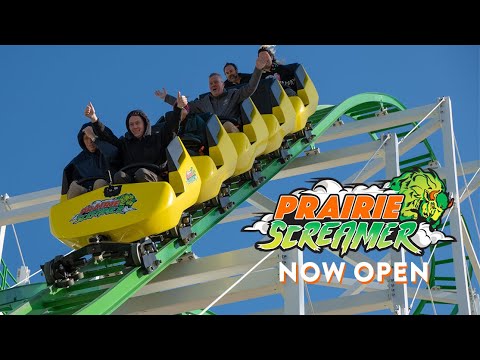The horizontal advertisement showcases a vibrant scene of the Prairie Screamer roller coaster, now open. The close-up image captures the exhilarating moment just as the coaster car begins its descent from the peak of the ride. The green-painted tracks and white supports stand out against the clear blue sky. The roller coaster car is vividly yellow, adorned with accents in green, white, and orange. Inside the car are several thrilled riders, some with their arms raised, grinning and screaming as they brace for the drop. Most of the passengers are men dressed in black shirts and dark tan pants, adding to the sense of unity and excitement. The image is bordered by two black bars, enhancing the focus on the center action. The advertisement text, "Prairie Screamer, now open," is superimposed in colorful, eye-catching fonts— "Prairie" in orange and "Screamer" from a darker to a lighter green—positioned on the right side, clearly marking the thrilling experience that awaits at this high-intensity amusement ride.